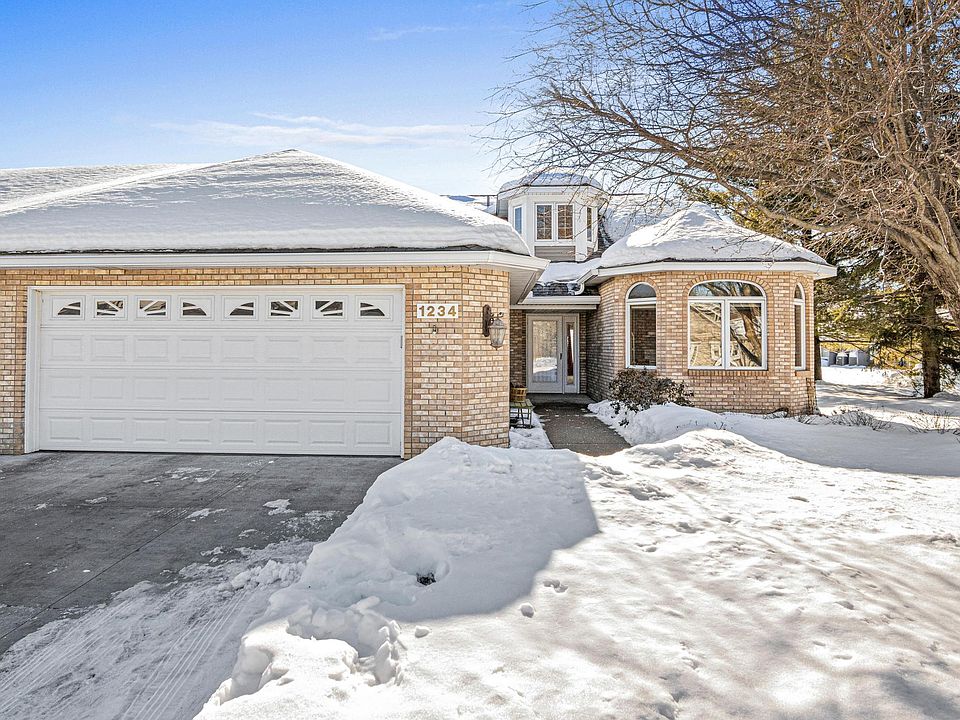This rectangular photograph depicts a serene winter scene featuring a tan and light brick two-story house with a snow-covered roof. Dominating the left side of the image is a big two-car garage with a white wooden door, positioned next to a lamp post. Above the garage, the house number "1234" is prominently displayed. The driveway, partially cleared of snow, stretches out in front of the garage, made of asphalt. A neatly shoveled sidewalk leads up to the front entrance, which boasts a white door. To the right of the entrance, there is a distinctive rounded room adorned with large picture windows. The entire property, including the grass and part of the driveway, is blanketed in snow. On the right side of the image stands a tall, barren tree, its leafless branches accentuating the wintry atmosphere. Further in the background, some trees with foliage can be seen. The sky above is mostly blue with a few clouds, adding to the tranquil ambiance of this outdoor scene.